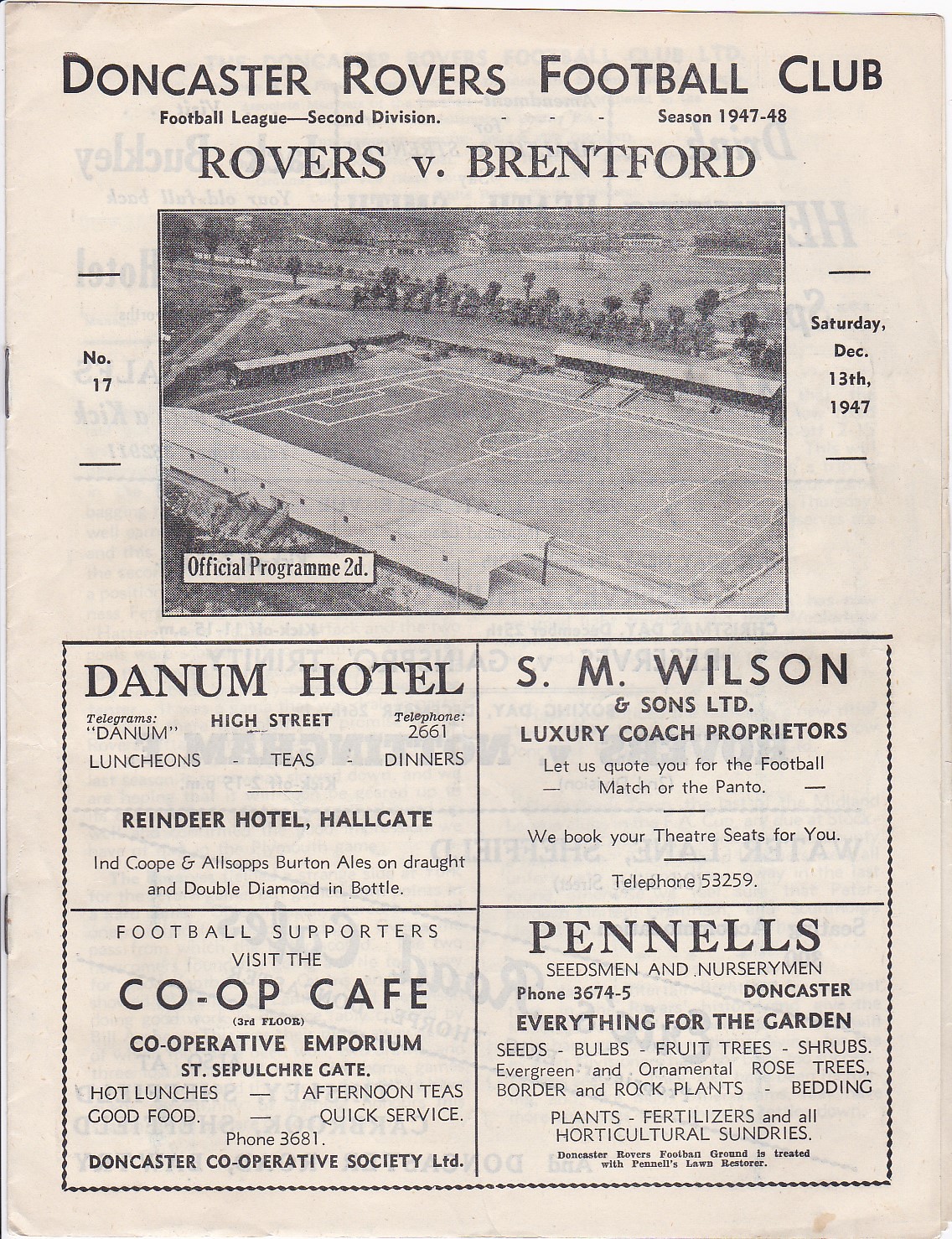The image depicts a vintage poster, seemingly a cover of a pamphlet or old magazine, advertising a football match for the Doncaster Rovers Football Club. The background is the cream-colored, slightly wrinkled, and stained paper typical of the era. At the very top, bold black letters announce "Doncaster Rovers Football Club." Below this, in smaller black font, it states "Football League, 2nd Division" and "Season 1947-48." Following this, in larger font, is "Rovers v. Brentford." 

Beneath the text is a black-and-white aerial photograph of an empty football pitch surrounded by trees and open fields, suggesting the image may have been taken from a height, perhaps from a helicopter. The bottom left corner of the photograph bears the inscription "Official Program 2D." Additionally, "No. 17" is written to the left, and "Saturday, Dec. 13, 1947" is on the right.

At the bottom of the poster are four rectangular advertisement boxes, outlined with a white and black dotted line. The left box advertises the "Danum Hotel, High Street." The next box to the right promotes "S.M. Wilson & Sons, LTD, Luxury Coach Proprietors." The bottom left box invites "Football Supporters" to the "Co-op Cafe, Cooperative Emporium." Finally, the bottom right box advertises "Pennell's, Seedsmen, and Nurserymen." Each advertisement contains smaller text with further details. All the text and images are rendered in black against the tan background of the newsprint.